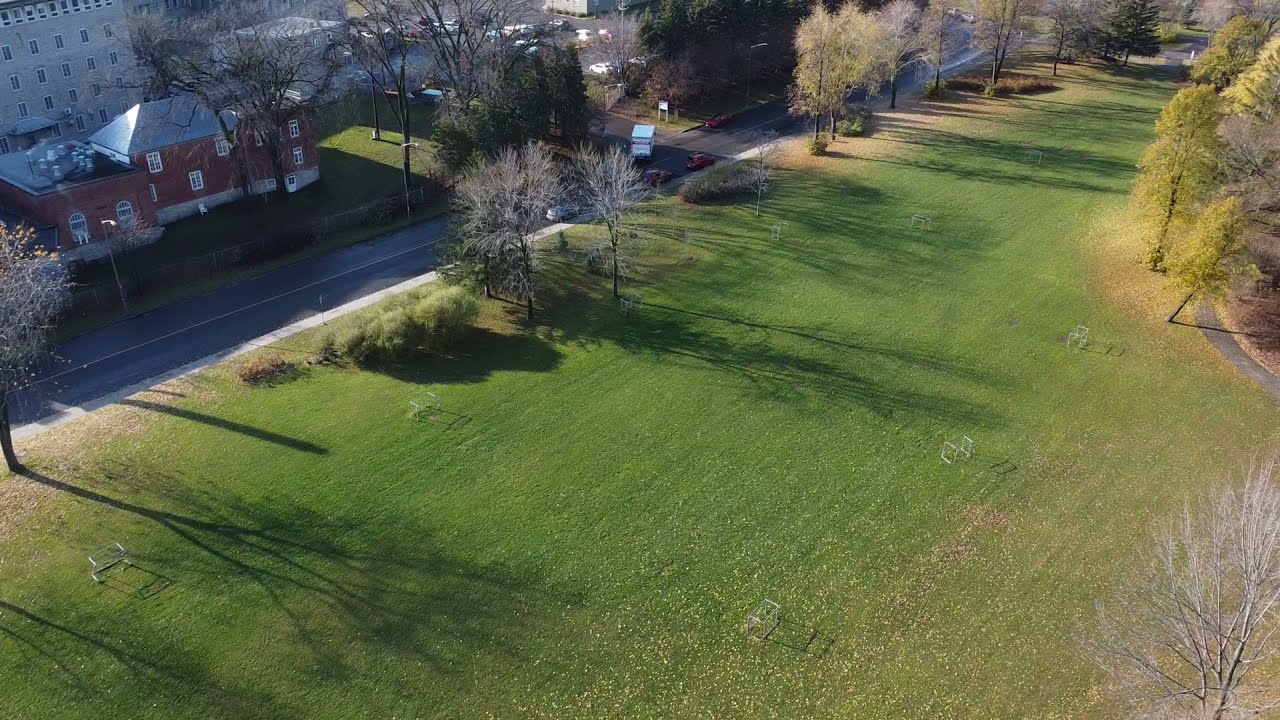This image is a brightly sunlit aerial photograph taken from above a park. The park, with its lush green grass and scattered fallen leaves, occupies most of the frame. It includes a few trees and shrubs, as well as benches and potential playing areas, with plants and trees of various sizes and types planted at regular intervals. To the left side of the park runs a two-lane street, where several cars and trucks can be seen in motion. On the opposite side of the street, there are a series of buildings. Prominently, there are two red brick buildings with white windows, possibly old campus or residential structures. Beyond these, there are taller multi-story office or residential buildings with silver-gray roofs. A parking lot filled with several cars, marked by a white entrance sign, lies adjacent to these buildings. The overall scene is void of people, emphasizing the serene atmosphere under the clear, sunny sky.